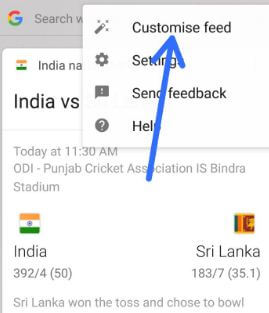The image depicts a search interface page with a prominent grayed-out Google logo positioned in the upper left-hand corner. Below this, a search bar features a partially visible query: "India VS." The screen provides detailed information about a cricket match scheduled today at 11:30 a.m. under the One Day International (ODI) format at the Punjab Cricket Association IS Bindra Stadium. 

The match score displays the Indian flag and the text "India 392/4 (50)," indicating India's score. To the right, the Sri Lankan flag is shown with "Sri Lanka 183/7 (35.1)," reflecting Sri Lanka's current standing. A note underneath states, "Sri Lanka won the toss and chose to bowl."

Additionally, there’s a pop-up with a blue arrow pointing towards the magic wand icon, which represents the custom feed option. Further down, standard navigation icons are present: a gear icon for settings, a speech bubble with an exclamation point for sending feedback, and a gray dot containing a white question mark for help.